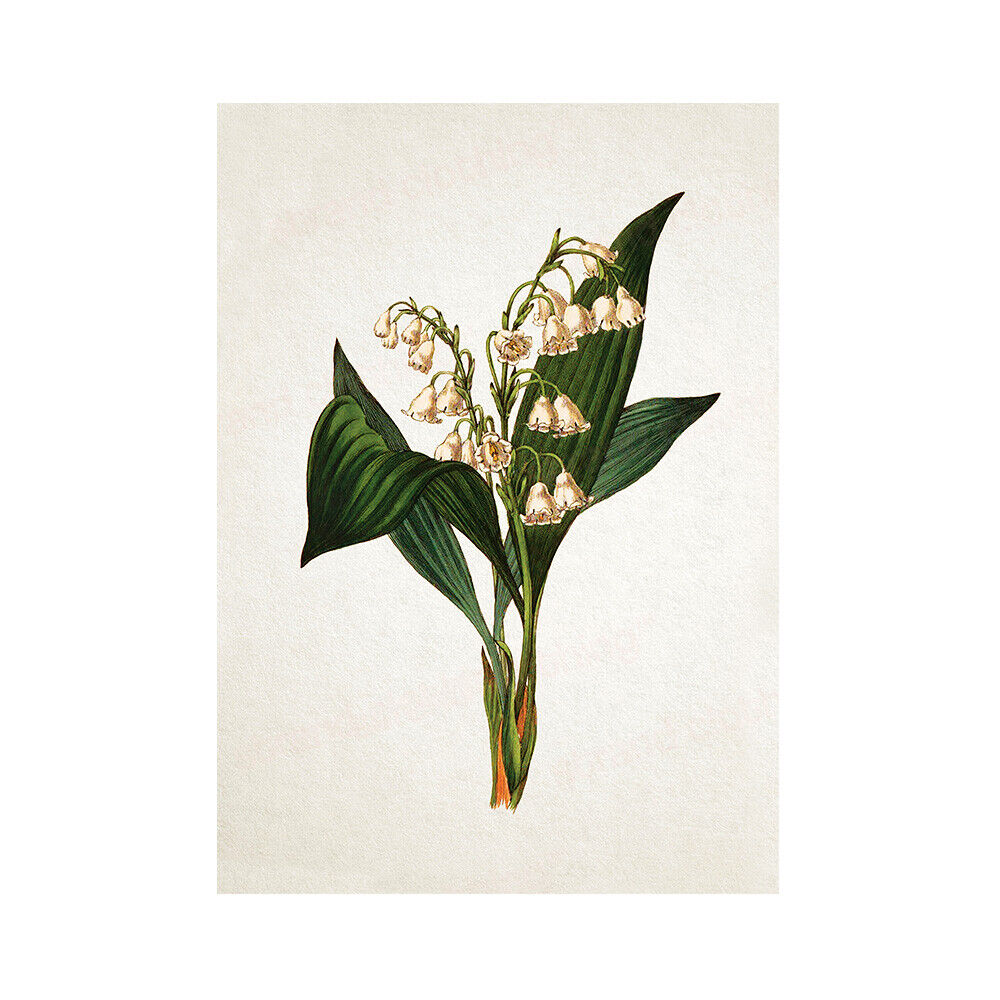The image is a detailed vintage illustration, reminiscent of 1800s European botany illustrations, of a lily of the valley in full bloom. The plant is drawn on a parchment-like background, which has a white color with a gray aura around the outer edges. The center of the plant features four tall, rich green leaves with unbranched vertical veins running from the leaf tips to the base. Nestled within these leaves are two green stems bearing a multitude of delicate, bulb-shaped white flowers, approximately 25 in total. Each flower droops downwards, resembling small, scalloped bells. The illustration stops at the green stem, showing some brown at the base where the leaves converge, and omitting the roots. The overall composition is simple and centrally focused, capturing the plant with fine ink lines and accurate colors.